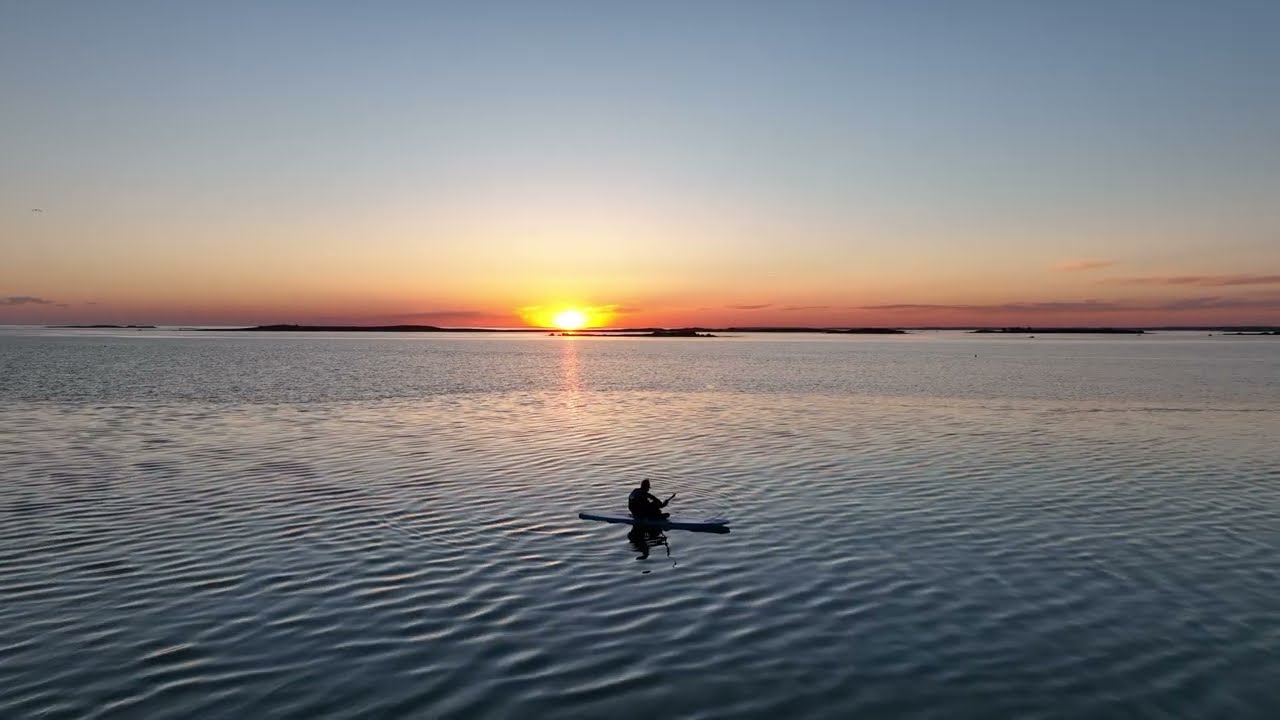The image is a stunning color photograph taken at sunset, featuring a silhouetted gentleman paddling a small kayak on a serene body of water, either a lake or ocean. Captured from a drone in landscape orientation, the scene portrays the man positioned towards the bottom center of the frame. The sky unfolds in a magnificent gradient, transitioning from dark blue at the top to gray, then to a peach and pinkish-red band near the horizon. A small white sun with a yellow glow hovers just above the water, casting a subtle light. The water is calm with gentle ripples, indicating a light breeze. In the background, narrow, rocky outcroppings also silhouetted by the setting sun create a beautiful contrast against the colorful sky.